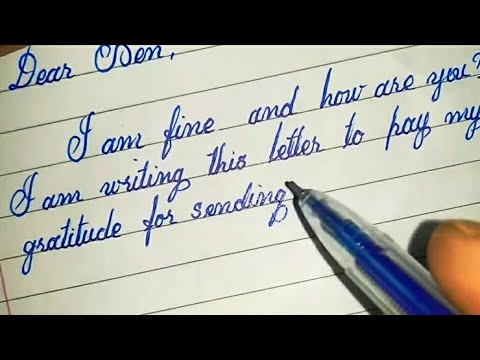The image appears to be a highly realistic rendering or photograph of a piece of white, lined notebook paper with cursive handwriting in blue ink. At the top of the paper, the text begins with "Dear [name]"—the exact name is difficult to discern but could be "Ben," "Jen," or "Dem." The content of the letter starts with "I am fine and how are you? I am writing this letter to pay my gratitude for sending," but it fades out as if the pen is running out of ink. The lines on the paper are black or gray, and we can see a clear blue-ink pen in the lower right corner, held by a finger with peach-colored skin. The pen is transparent, revealing its blue ink cartridge, and has a yellowish point. The background is partly black at the top and bottom with a small tan desk visible behind the page. The overall scene captures the intimate moment of someone writing a heartfelt letter.